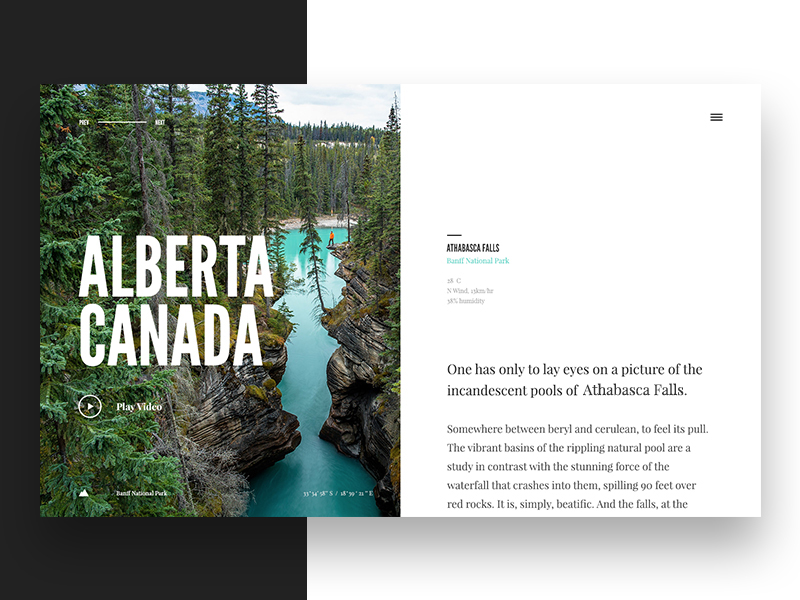A detailed caption:

The image showcases a screenshot of a computer page with a distinct layout. On the left side, there is a prominent black vertical rectangle, while the rest of the screen is white. Dominating the center is a large white rectangular area, overlaid by a pop-up box. The left half of the pop-up features a stunning outdoor photograph depicting a serene river flowing amidst rugged cliffs, with bright turquoise water that exudes clarity and vibrance. The captivating scene is set in Alberta, Canada, highlighted by bold white text. A lush forest of fir and evergreen trees surrounds the river, with majestic mountains rising in the background.

Below the title, there's an option to play a video. On the right side of the pop-up, the name of the falls (beginning with an A) and "Banff National Park" are displayed in turquoise text, followed by brief, smaller text providing additional details. The article beneath the pop-up describes the breathtaking beauty of the pools at Athabasca Falls, stating, "One has only to lay eyes on a picture of the incandescent pools of Athabasca Falls," with further information about this picturesque location. In the distance, a man in a red shirt can be discerned, adding a human element to the natural splendor.